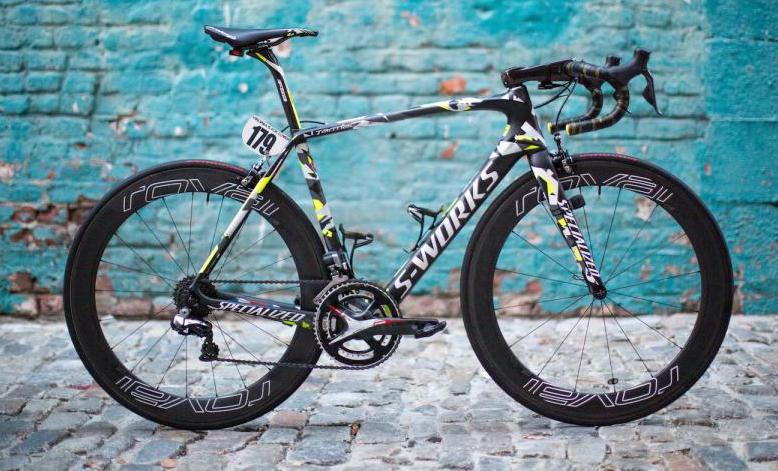The image is a detailed color photograph of a high-performance racing bicycle, evidently designed for marathon riding. The bike features characteristic forward-curving, upside-down handlebars akin to those found on a 10-speed model, with the brakes mounted on the front. Its frame is predominantly black with prominent white "S-Works" branding near the handlebar stem. The black racing tires are set against this frame, hinting at the bike's specialized construction. The seat is positioned high and is black, complemented by small yellow and white stripes near it and other parts of the bike. Notably, a tag with the number 179 is attached behind the seat, suggesting a race identifier. The bicycle is situated on a cobblestone path with varying shades of gray. The background reveals a weathered teal or turquoise brick wall with sections of exposed red brick, providing a rustic and contrasting setting for the sleek bike. The wider image appears to be a product photo captured in a natural, outdoor environment.